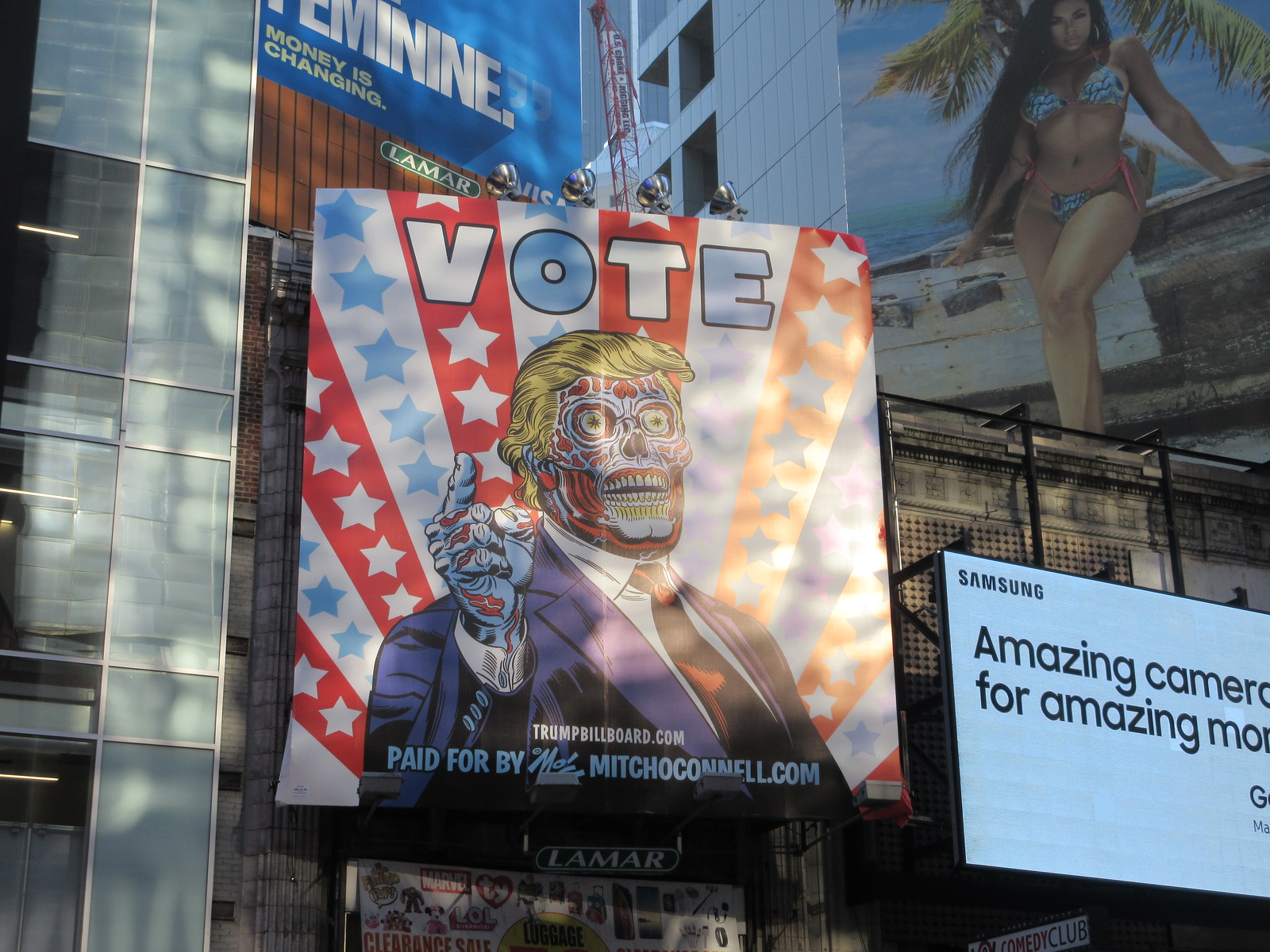In the bustling cityscape dominated by towering skyscrapers, a series of striking billboards demand attention. The centerpiece is a vivid and controversial billboard featuring an artistic rendition of Donald Trump, portrayed in a sugar skull style with exposed veins and muscles, giving his face a skeletal appearance. The image is adorned with red and blue stripes and stars, with Trump pointing forward in a blue-suited arm. Boldly, the word "VOTE" is emblazoned above this grotesque caricature, and a URL, trumpbillboard.com, is promoted, noting that it’s paid for by mitchmcconnell.com, alongside the initials "MOC."

Flanking this dominant image, additional billboards reflect the diverse vibrancy of city advertising. Below Trump's billboard, a storefront advertises a clearance sale featuring Marvel and Beanie Babies merchandise. Above it, another sign declares, "Feminine money is changing." To the right, a glamorous billboard showcases a woman in a bikini beside a palm tree, evoking a beachy allure. In the lower right corner, a sleek digital Samsung advertisement boasts, "Amazing camera for amazing moments," though the full text is partially obscured.